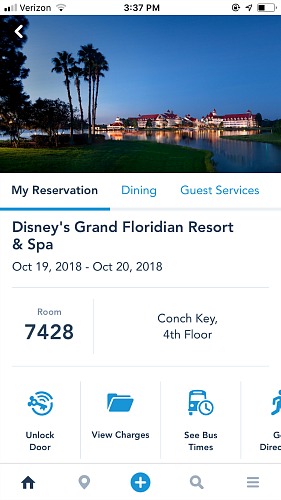The image displays a smartphone screen showing a webpage from Verizon. At the top, there are indicators for cellular signal, Wi-Fi signal, and the time reads 3:37 PM. To the right, there are icons for an arrow, a lock, and a half-filled battery.

The center of the screen contains a graphic of an outdoor scene, portraying a sky transitioning from dusk to night with darker blue hues. The landscape features an array of trees, including palm trees and taller varieties, a body of water, and a distant backdrop of what appear to be hotels. The foreground is adorned with grass.

Below the graphic, on a white background, the text "My Reservation" is underlined with a blue line. Blue text beneath it reads "Dining and Guest Services." Further down, it provides details of a reservation at Disney's Grand Floridian Resort and Spa, spanning from October 19, 2018, to October 20, 2018, for room 7428 in the Conch Key building, on the fourth floor.

At the bottom, there are icons representing various options and tools: "Unlocked Door," "View Changes," and "See Bus Times," with another icon that is blocked out. Additionally, there are icons for a home, location, a blue circle with a plus sign, a magnifying glass, and a stack of three gray horizontal lines.